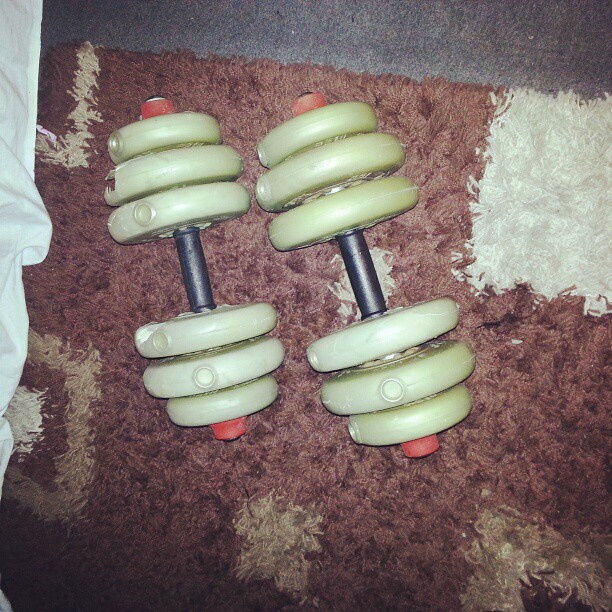This photograph captures an aerial view of two dumbbells resting on a shaggy, multicolored carpet. The primary carpet color seems to be a mix of brown, white, and rusty reddish-orange, featuring a pattern that includes white and gold squares. Each dumbbell consists of a black central bar flanked by three weights on each end, arranged from larger in the middle to smaller on the outside. The weights themselves are light green, and the dumbbells are capped with bright orange ends. One dumbbell leans slightly towards the other. On the left side of the image, part of a white material—possibly a table skirt or bedspread—is visible. In the upper part of the image, part of the original floor, which appears to be gray tile or cement, can be seen beneath the rug. The exact weight of the dumbbells is not specified.